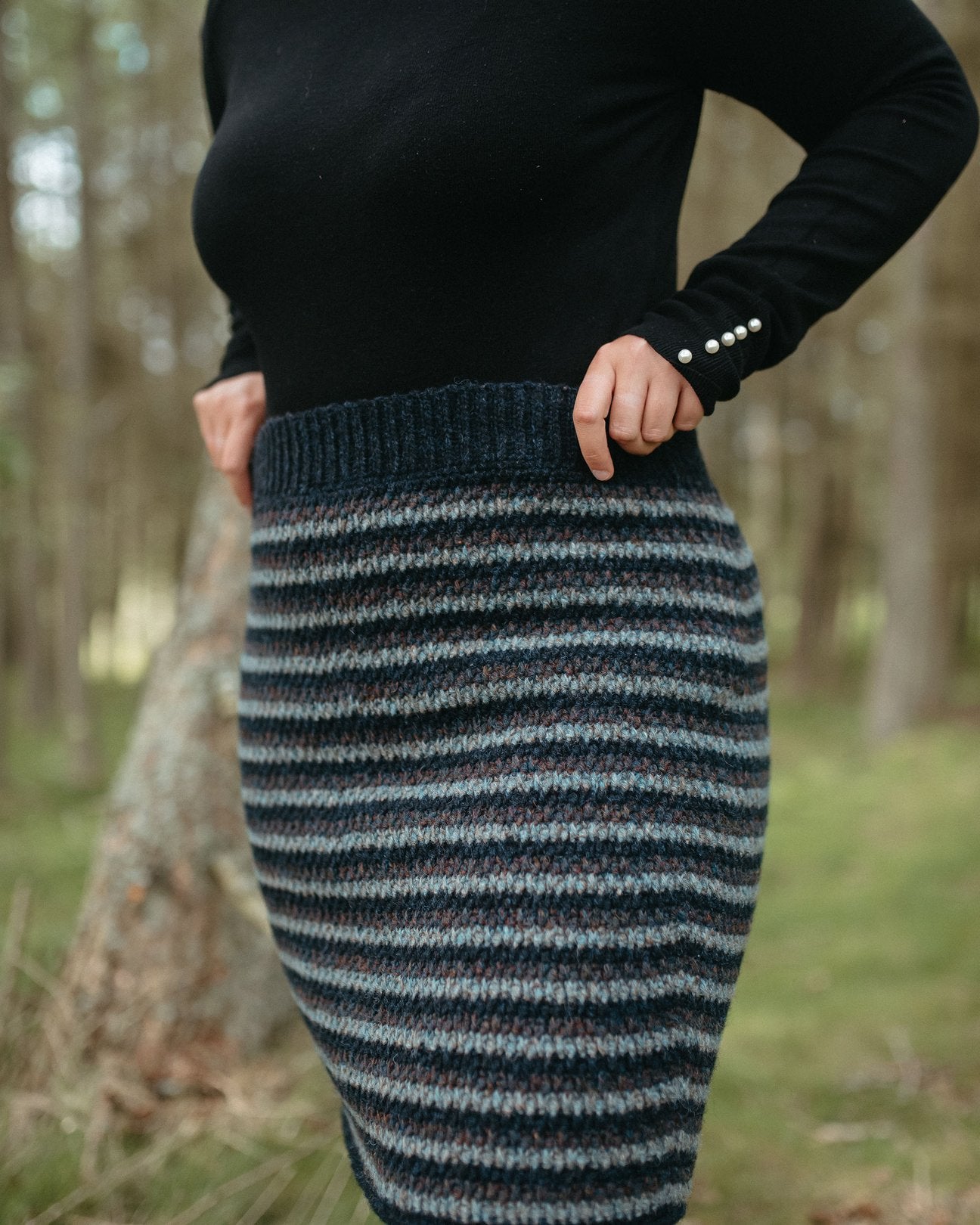The photograph depicts a close-up view of a woman's outfit, framed from her shoulders down to her knees. She is wearing a black, long-sleeved sweater adorned with five pearl buttons on each cuff. Her hands, devoid of rings, rest near the waistband of her knitted skirt, which features a pattern of thin, alternating stripes in dark gray, light gray, and black. The top waistband of the skirt is distinctly dark gray. In the blurred background, one can discern trees and grass, suggesting an outdoor setting. To the left of the woman, there's a visible tree stump positioned closer to the foreground. The composition emphasizes the intricate details of her attire against a natural, slightly out-of-focus backdrop.